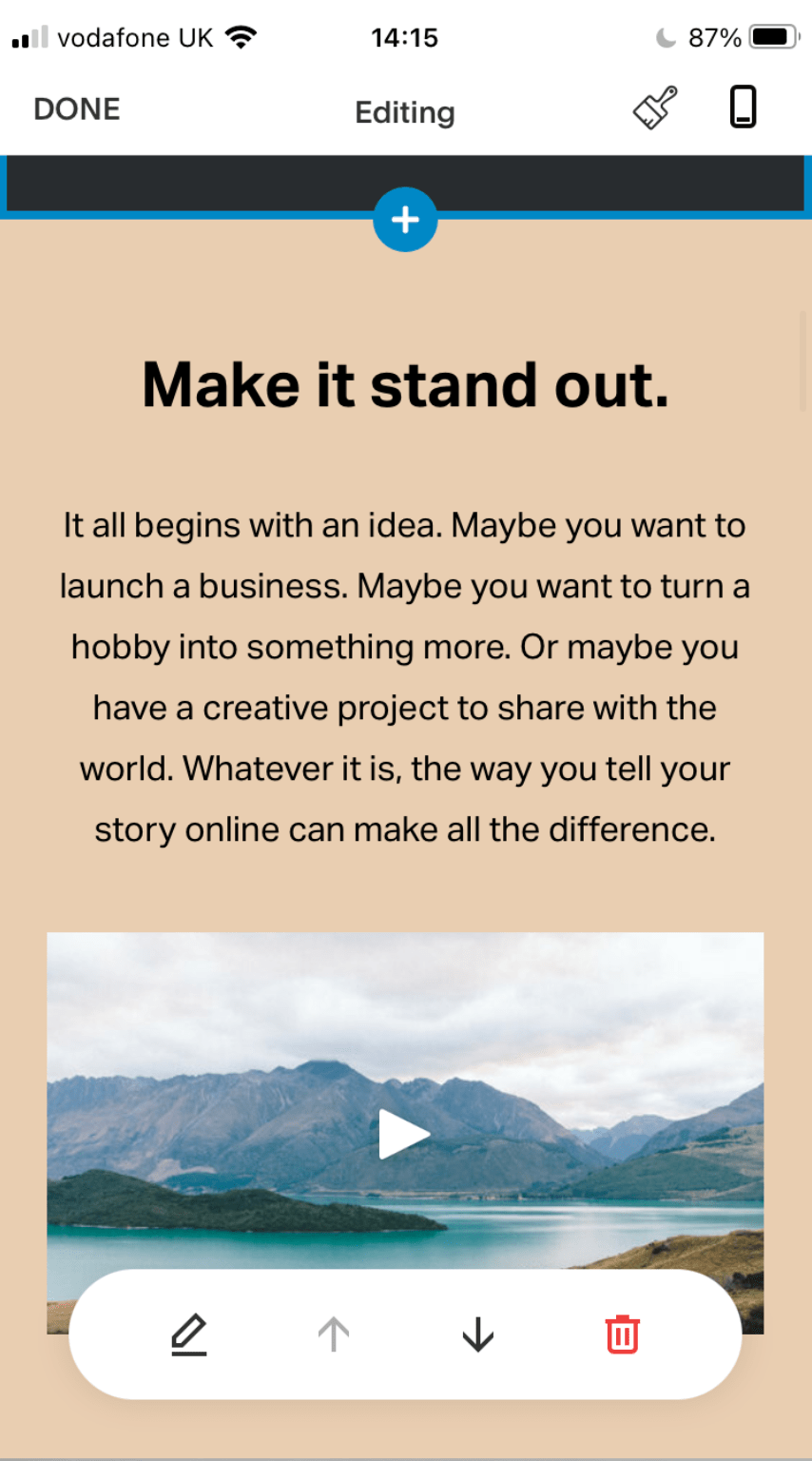This image appears to be a screenshot taken from a mobile device, showcasing a webpage or app. At the top of the screen, the status bar indicates "Vodafone UK" as the carrier, with the time displayed as 14:15. Next to the time, there is a moon icon and a battery life indicator showing 87% remaining. Below the status bar, the text "DONE" is written in large, black, capital letters, suggesting the user has completed editing. 

The editing tools visible include a paintbrush icon and a cellphone icon, hinting at customization or design options. The central portion of the screen features a paragraph with the heading "MAKE IT STAND OUT" followed by a plus sign that signifies an option to add more content. The paragraph reads: "It all begins with an idea. Maybe you want to launch a business, maybe you want to turn a hobby into something more, or maybe you have a creative project to share with the world. Whatever it is, the way you tell your story online can make a difference."

Towards the bottom of the screen, there is a video placeholder with a play button, indicated by a triangle pointing to the right. The background of the video preview shows a scenic view of mountains and a lake with beautiful, clear water. Finally, several icons are visible at the very bottom of the screen, likely representing various navigation or action options.